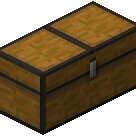The image depicts a computer-generated wooden chest, resembling the design of a Minecraft chest. The chest is rendered in varying shades of brown, with the top portion being a lighter hue compared to the sides, which are slightly darker. It has distinctive black lining that runs along its edges, including the strap-like features that wrap over the top and down the sides. The chest appears to be viewed from a three-quarters angle, allowing visibility of the top, front, and right side. The front of the chest features a silver-grey metal latch used for locking it, and the top is divided by trim into two squares. Notably, parts of the chest on the right and left sides are cut off, reinforcing the computer-animated nature with minor pixelation. The trunk sits against a white background, emphasizing the contrast of its detailed texture and colors.